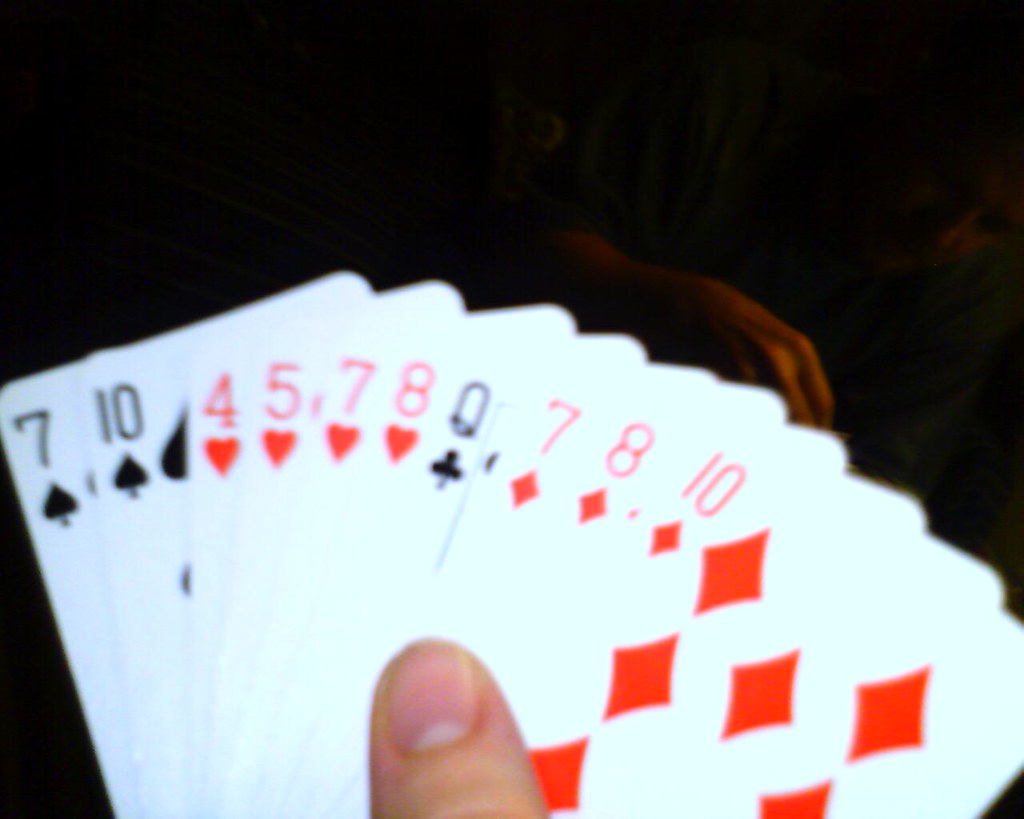In the image, a hand of playing cards is prominently displayed against a pitch-black background, adding a dramatic depth to the scene. The partial view of the hand, with just the thumb visible holding the cards, suggests an intense moment in a poker game. The thumb holds the cards at the front while the other fingers are presumably hidden behind the spread. 

The card hand appears to be exceptionally strong, featuring a sequence of key cards: three sevens (from clubs, hearts, and diamonds) and a pair of tens (from clubs and diamonds). The specific arrangement of the cards from left to right includes: the seven and ten of clubs, the seven and eight of hearts, the queen of clubs, and the seven, eight, and ten of diamonds. A notable ten is also present in this ensemble. The cards are simplistic in design—entirely white with standard print for the suits and numbers located at the top, lacking any ornate or decorative elements.

The meticulous arrangement by suit and the clear depiction of the cards' values and suits amplify the focus on the impressive hand being held, likely eliciting anticipation of a favorable outcome in the game.